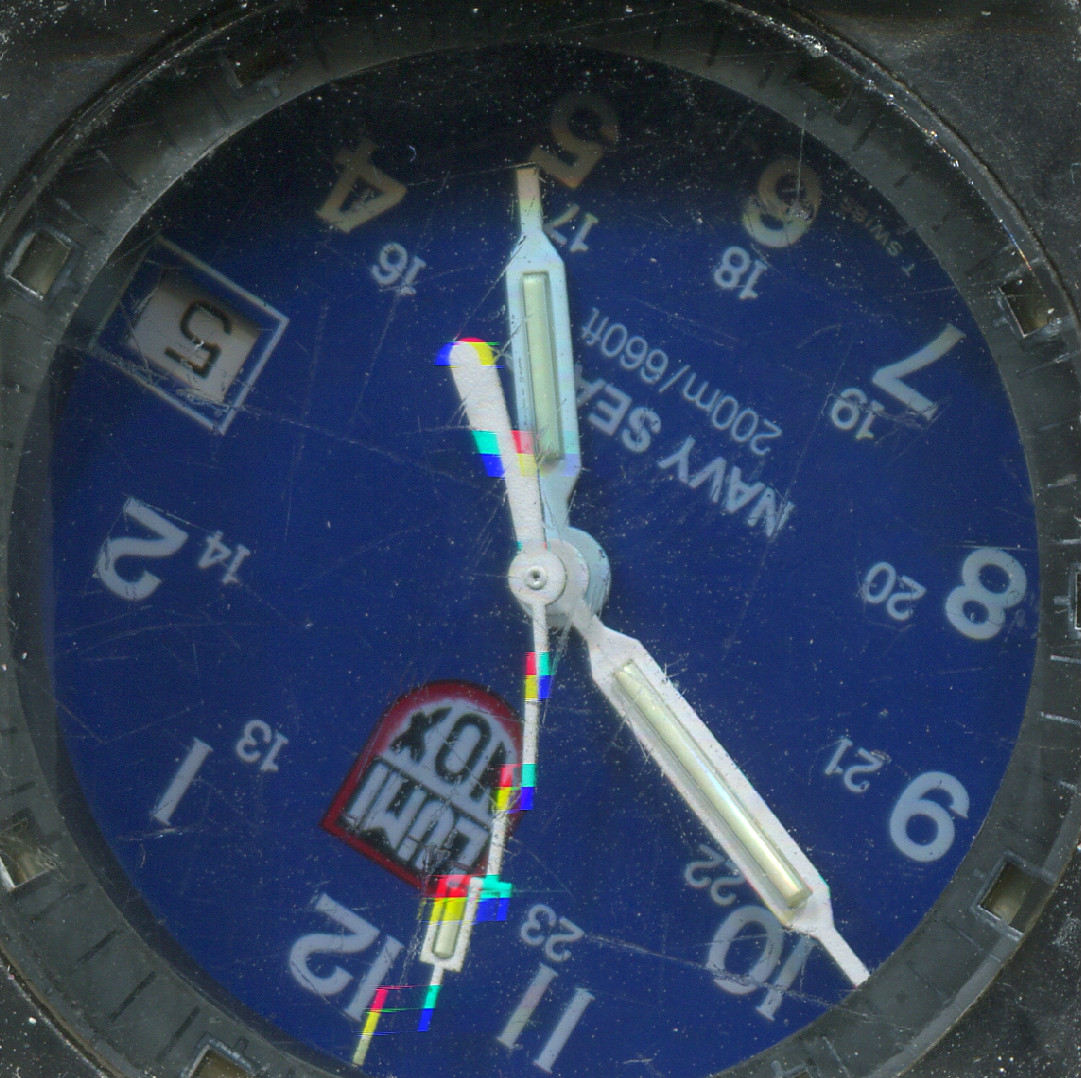An up-close, detailed image of a watch face, shown upside down. The rich blue face contrasts with its polished silver casing, though the watch band is not visible due to the tight framing of the shot. The white numerals marking 12, 1, 2, 4, 5, 6, 7, 8, 9, 10, and 11 stand out distinctly against the blue background, while the number 3 position houses a date display showing the 5th. The hour, minute, and second hands are all white, providing clear visibility. At the center of the watch face, the brand name "Luminox" is prominently displayed in the middle with a red border on a black and white background. The watch boasts its durable waterproof capability, rated at 200 meters or 660 feet, with "Navy Seal" inscribed to highlight its robust features.